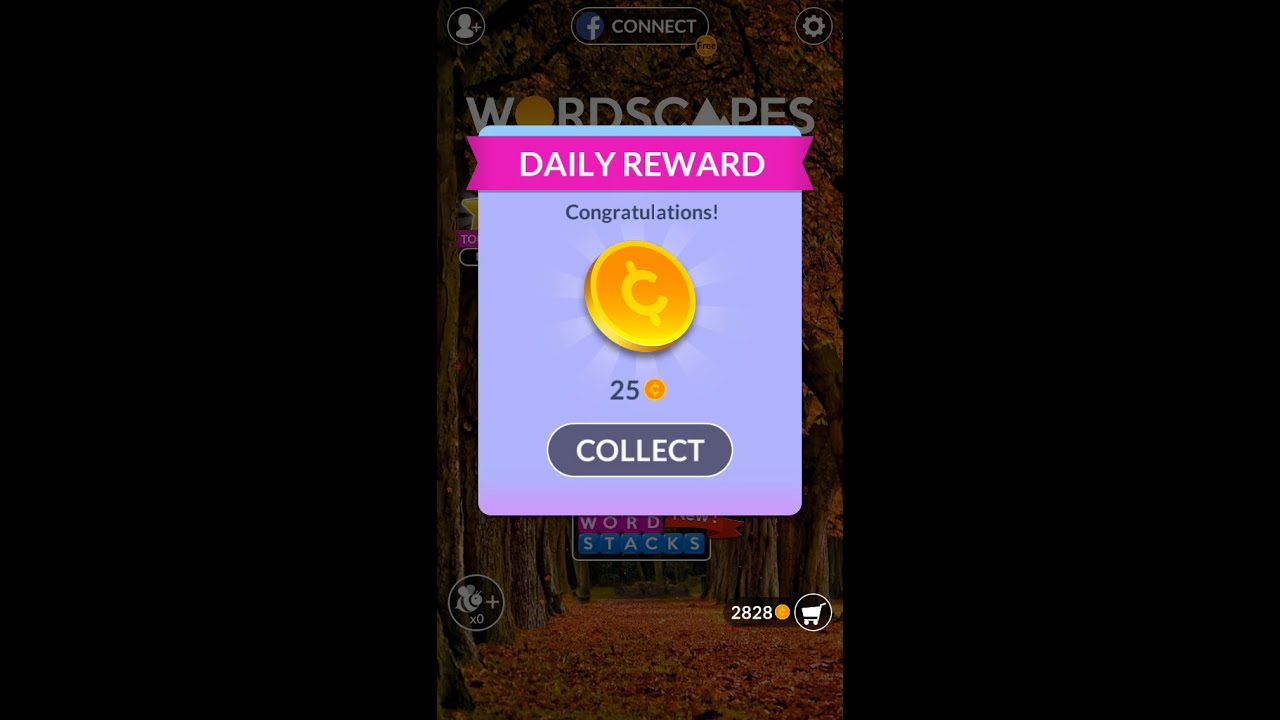The image is a detailed screenshot from the mobile game Wordscapes, featuring a vibrant autumnal background of tree-lined streets with orange, yellow, and brown leaves covering the ground. In the foreground, a prominent pop-up notification with a vivid pink and purple design displays the text "Daily Reward" in bold white letters with a pink banner beneath it. Directly under this banner, the word "Congratulations" appears in black font, followed by a shining gold coin illustration with a cent symbol and the number "25" below it. The pop-up is completed with a button labeled "Collect."

At the bottom left of the main screen, there is a 'B' with a plus sign enclosed in a circle, while to its right, the screen displays a total of 2828 coins alongside a shopping cart icon. The top left features an icon for adding a friend, and the top center shows a Facebook Connect button prominently displayed with the Facebook logo and a "free" coin offer. On the top right, there is a settings button.